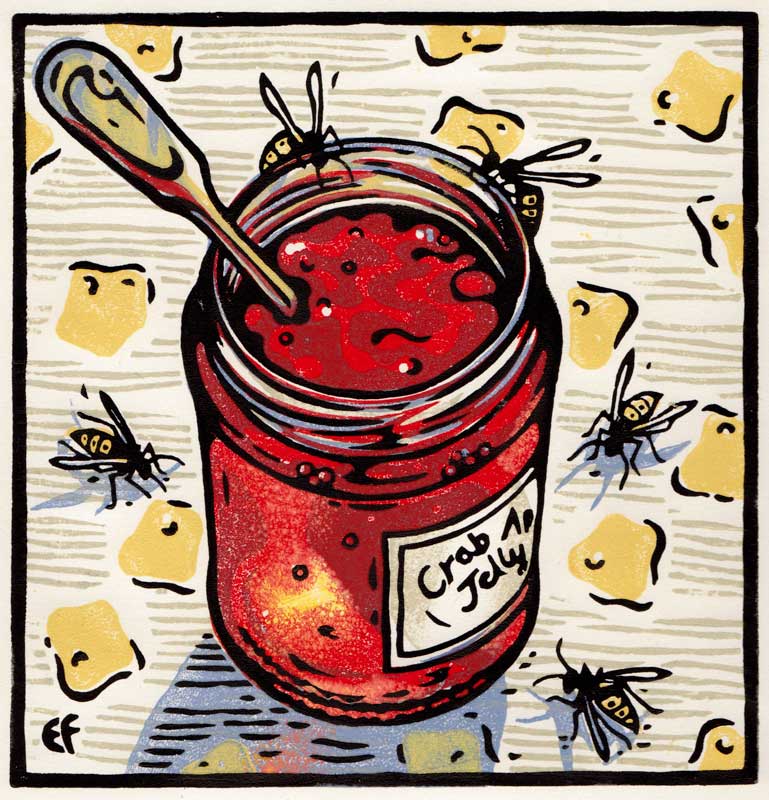This illustration depicts a crystal-clear jar filled with vibrant red crab apple jelly. The white label on the side of the jar clearly reads "Crab Apple Jelly" in black font, though only part of the text is fully visible. Emerging from the top left of the lidless jar is a utensil, likely a spoon, though its base is obscured. The jelly itself is depicted with red bubbles and dark red swirls inside, adding texture and richness to the vibrant red color. Surrounding the jar are various elements on a wooden table, evidenced by horizontal brown stripes. Five bee-like creatures or wasps with yellow stingers and black bodies are also present; two are climbing up the jar, near the lip where the cap would go, while three are on the table, alongside what appear to be pieces of cheese, yellow with a hole or two in them. The background features yellow splotches edged in black, perhaps representing honeycombs. The initials "EF" can be seen in the bottom left corner, indicating the artist's signature.